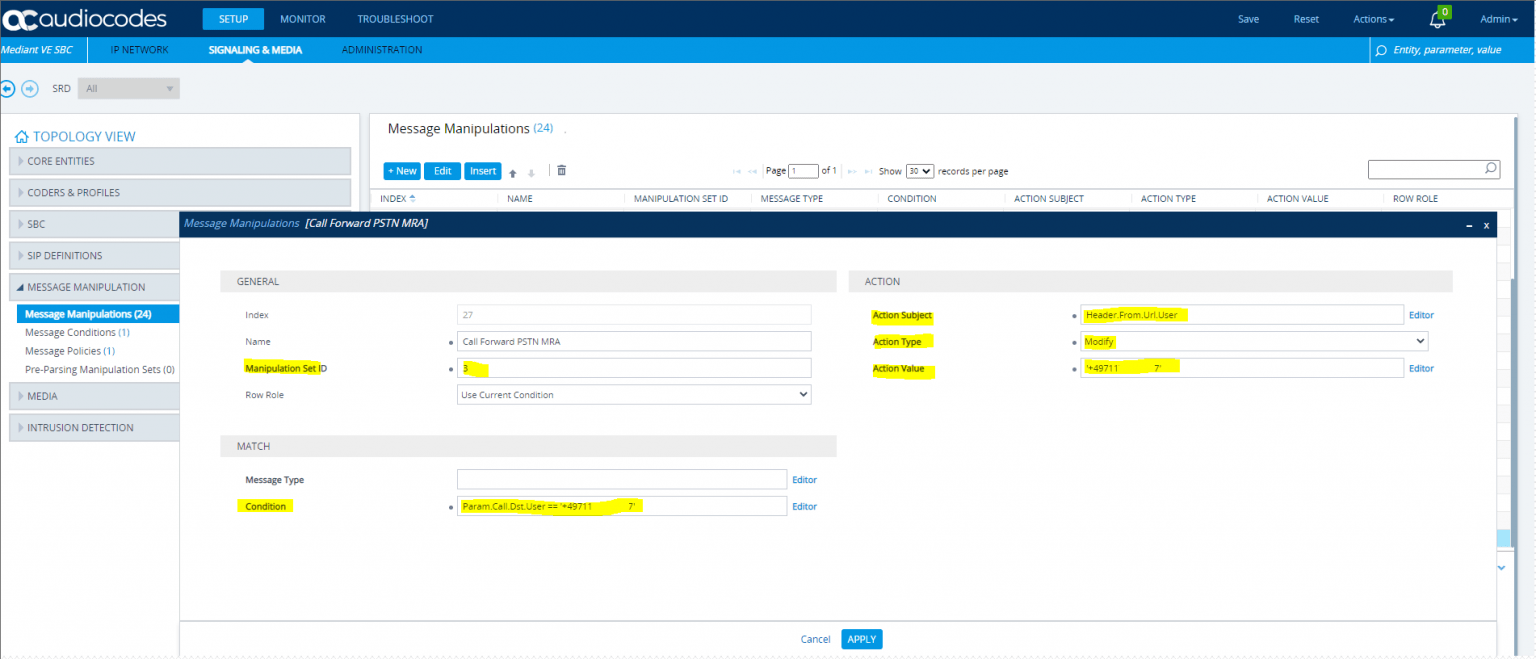This screenshot of a computer page from OC Audio Codes showcases a multi-layered layout with distinct color-coded sections. At the top, there is a dark blue strip featuring a notification alert in the form of a green box with a number inside. Beneath this, a lighter blue strip is visible, followed by a gray strip. The interface includes various small text options, which are difficult to read due to the text size.

In the top dark blue section, a notification icon can be seen, implying the presence of an alert or message. Directly below, a white box is prominently displayed, labeled "Topics OGY View," listing different topics within gray boxes. Another primary white section labeled "Message" includes what appears to be related information, possibly titled "Manufacturer's Map," although the small font renders it unreadable.

Additionally, there is a dark blue pop-up window on the page, characterized by numerous sections highlighted in yellow. This pop-up contains several fields for inputting information, with the highlighter marking specific areas throughout the form. The yellow highlights dominate the pop-up, indicating important areas of focus.